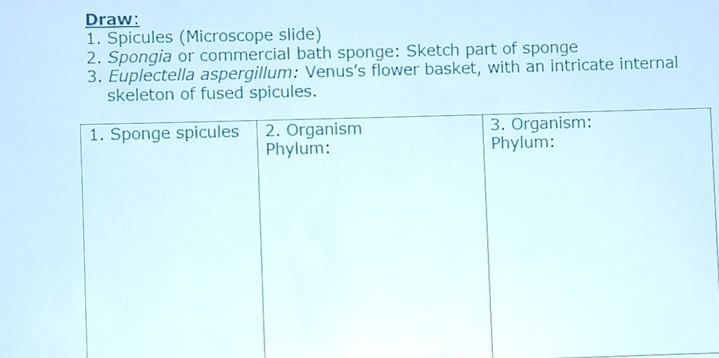This is a detailed photograph of a light blue piece of paper, likely intended for scientific use, possibly in a work or educational setting. At the top left corner, the word "draw" is underlined and followed by a colon. Below this heading, there are three numbered instructions. The first instruction reads: "1. Spicules (microscope slide)." The second instructs: "2. Spongia or commercial bath sponge: Sketch part of the sponge." The third details: "3. Euplectella aspergillum: Venus's flower basket with an intricate internal skeleton of fused spicules." Under these instructions, there are three empty boxes for responses. Box number one is labeled for "sponge spicules," and both box number two and box number three are labeled "organism phylum." This empty form, evidently awaiting completion, appears to be a worksheet or examination page, likely to be filled out by a scientist or student in the relevant field.